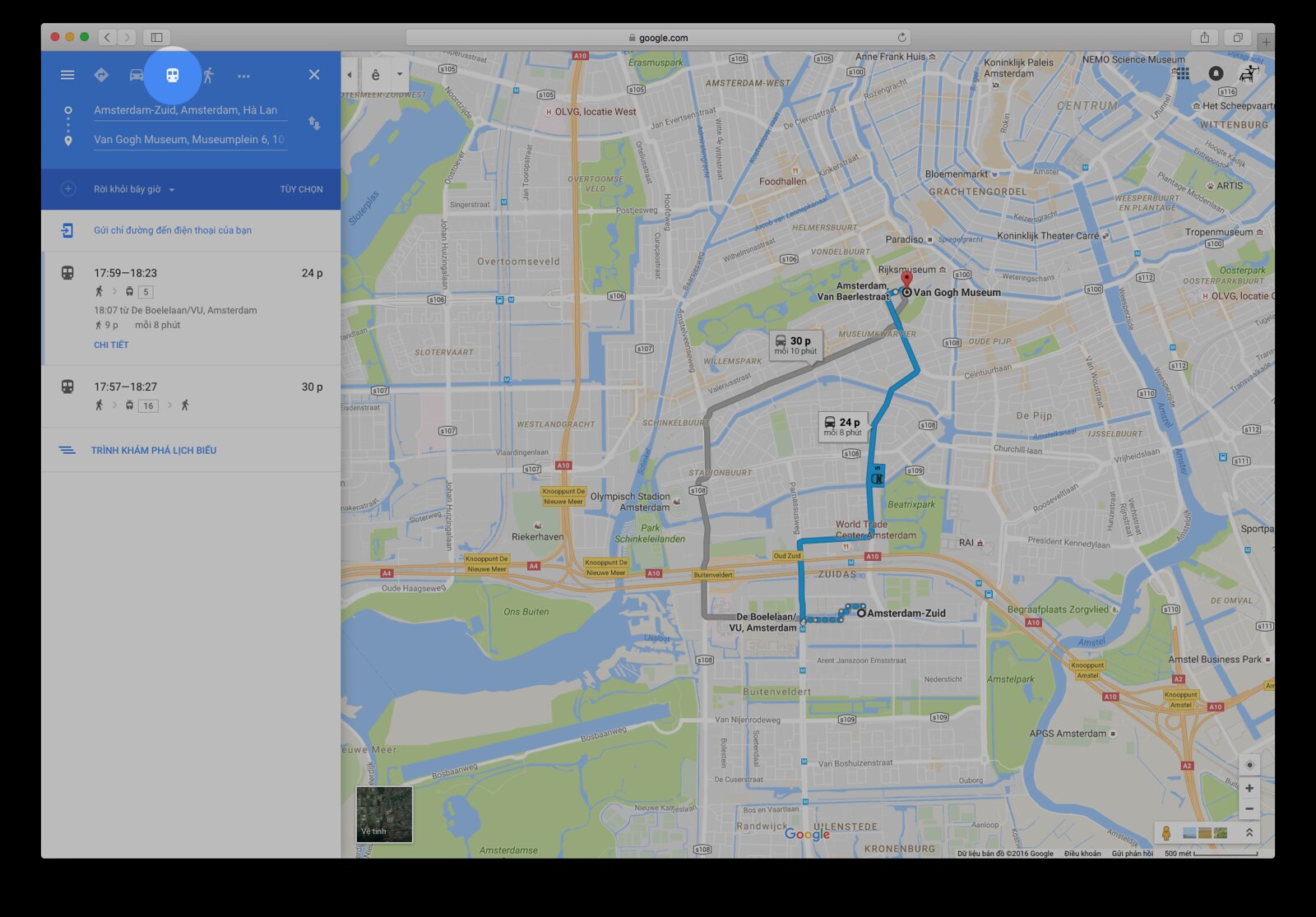**Descriptive Caption**

The image appears to be a screenshot from a Mac or Apple device, characterized by its prominent black border, which is thinner at the top and equally wide on the sides, but significantly larger at the bottom. Within the screenshot, a gray bar spans horizontally across the top. On the left side of this bar are three colored circles: red, yellow, and green. 

Adjacent to these, starting from the left, there's a sequence of light gray boxes each featuring different icons: a black arrow pointing left, a white arrow pointing right on a gray background, an icon resembling a book, a black arrow pointing upward within a black box, and a plain black square. 

Below this toolbar, the main content displays what seems to be a navigation interface, likely from a map application such as Google Maps. The left portion of the map features a transition from light blue to dark blue, interspersed with white areas. It includes navigation details specifying a route from a location in Amsterdam to the Van Gogh Museum. The routes are categorized based on travel options, showing transit times of 24 minutes by bus and 30 minutes by train. 

The map further illustrates a combination of geographic features and urban layouts: blue regions indicating lakes and rivers (more prevalent on the right side), yellow-marked major roads and highways, and smaller white streets with black text for names. Two possible routes are highlighted, with the most efficient one depicted in blue and the alternative in gray.